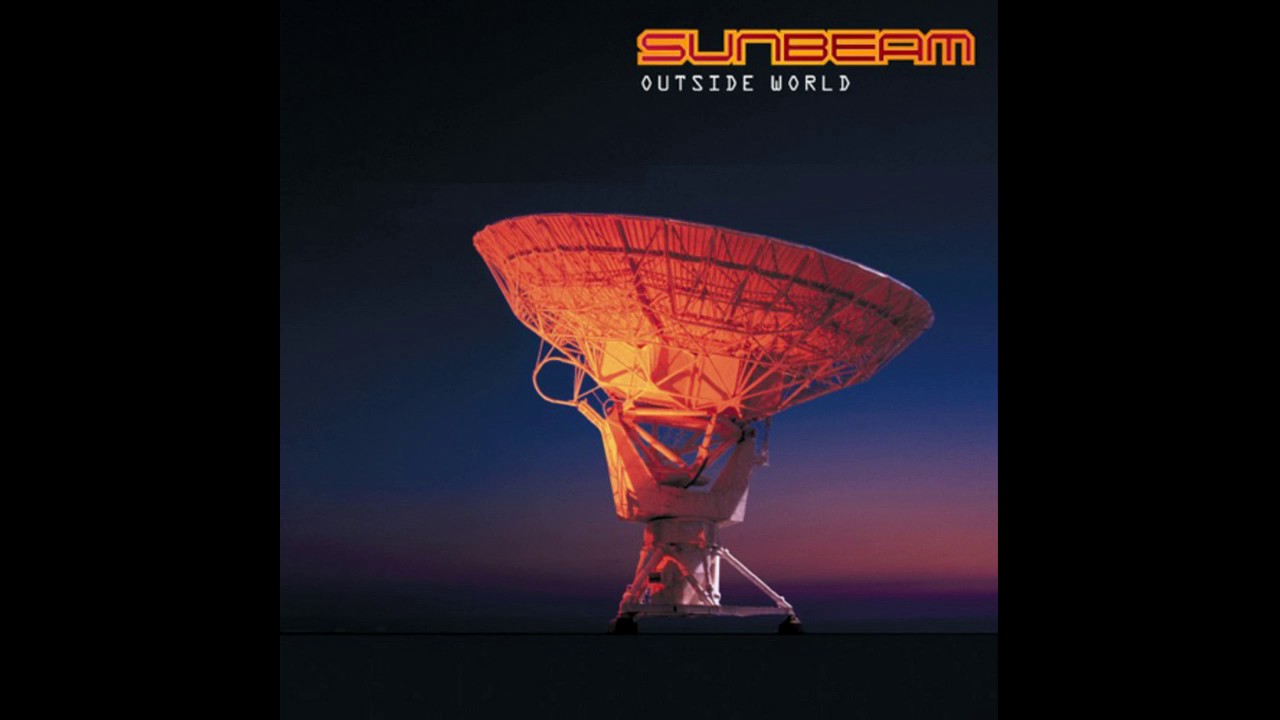The image depicts a large, white satellite dish centrally positioned against a black background. The dish, seemingly designed for space observation, is illuminated by a subtle red lighting. The backdrop features a dramatic, multicolored sky transitioning from black at the top to dark and deep blues, purples, pinks, oranges, and reds towards the horizon, suggesting either dawn or dusk. The satellite is positioned on dark-colored ground, enhancing the contrast with the vivid sky. In the upper right corner, bold red text with a white outline spells "Sunbeam," while directly beneath it, in plain white font, are the words "Outside World." The overall presentation, including the thick black borders on the sides and the nostalgic text style, hints that this might be a cover for a CD or a book.